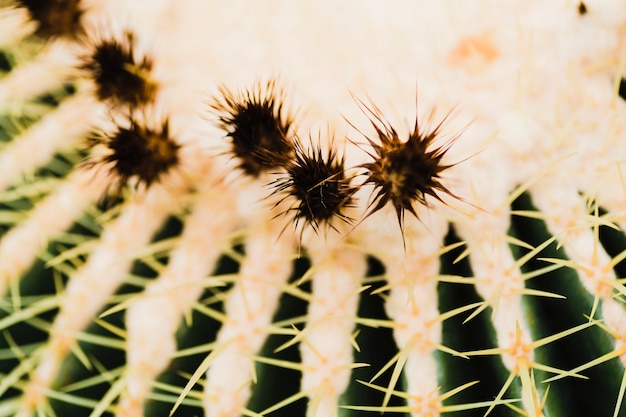This image presents a close-up view of a plant, likely magnified significantly, capturing intricate details of its structure. The dominant feature is a large white plant situated in the background, which is adorned with numerous spines radiating from its center. Surrounding this are several smaller plants or seedling structures, each characterized by black, spiky balls or spines. The green hue permeates the background, creating a glowing effect around the large white plant. These spikes resemble the types of thorny parts that commonly adhere to socks and shoes. The detailed view suggests a possibly microscopic perspective, emphasizing the textural and structural intricacies of what might be everyday yard vegetation. The image is primarily composed of whites, greens, blacks, and yellows, contributing to its vivid and meticulous depiction of the plant's spiny nature.